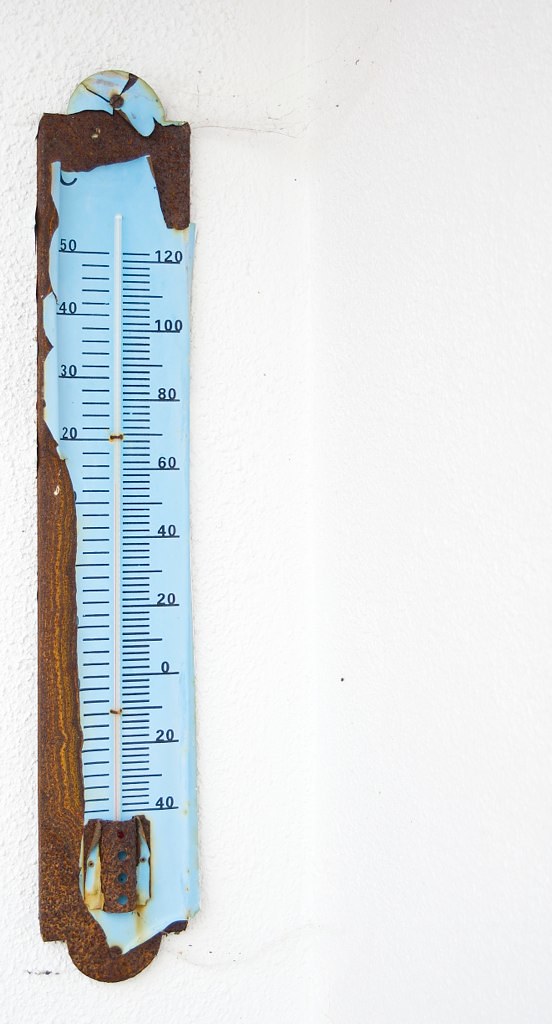The image features an antique thermometer affixed to a white wall, prominently positioned on the left side of the frame. The thermometer itself is predominantly blue, with significant rust accumulation along the left, bottom, and top edges, and a smaller patch of rust along the upper right edge. This rust, indicative of prolonged exposure to the elements, obscures the base and suggests that the thermometer was once secured by nails, visible through the four holes in the rusty section.

The thermometer presents dual temperature scales: Celsius on the left and Fahrenheit on the right. The Celsius scale appears incomplete, only showing values of 50, 40, 30, and 20 at the top before being cut off. In contrast, the Fahrenheit scale is fully intact, displaying a range from -40 up to 120, in 20-degree increments.

Notably, the thermometer lacks any fluid inside its glass tube, suggesting it is no longer functional, possibly broken. Despite its condition, the clear glass reveals the internal components and old craftsmanship. The bright, daytime setting highlights the age and wear of this once-functional instrument, capturing a sense of nostalgia and history.